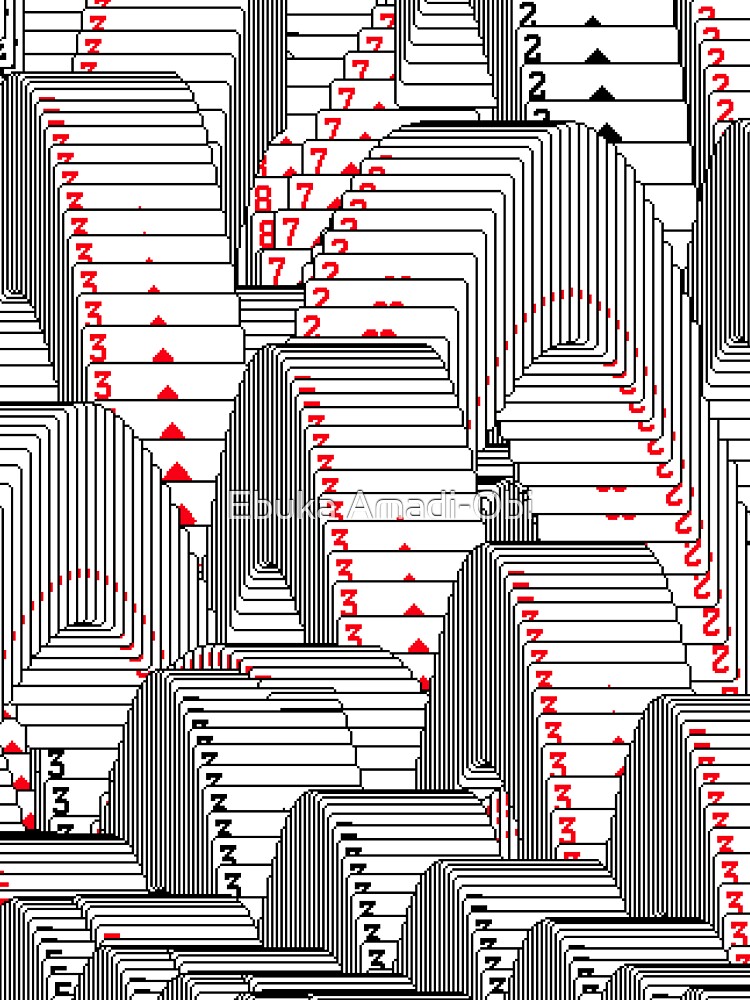This is a vibrant, clip art-generated image that nostalgically recreates an old-school screensaver, typically seen after winning a game of solitaire. The entire scene is filled with numerous archways, each composed of multiple playing cards repeatedly stacked to form grand, bridge-like structures. Dominating the foreground and background are arches made from the three of diamonds, each meticulously layered to create a cascading effect. Interspersed within these, black threes stand out prominently, with at least four visible archways of spades.

The image is richly detailed, featuring seemingly three-dimensional arches that give the illusion of cards jumping across the screen. At the top of the screen, rows of red sevens and red twos intersect in patterns, adding a lively variety. The top left corner houses a sequence of black threes, while the right side showcases both black and red twos in intricate formations.

Smaller clusters of the two of hearts and additional three of diamonds appear scattered throughout, emphasizing the randomness and playful chaos of the composition. The palette is strictly black, white, and red, which enhances the visual impact of the card arches. Overall, the image conveys a sense of dynamic motion and nostalgic charm, with cards forming elaborate tunnel-bridge structures that seemingly leap off the page.